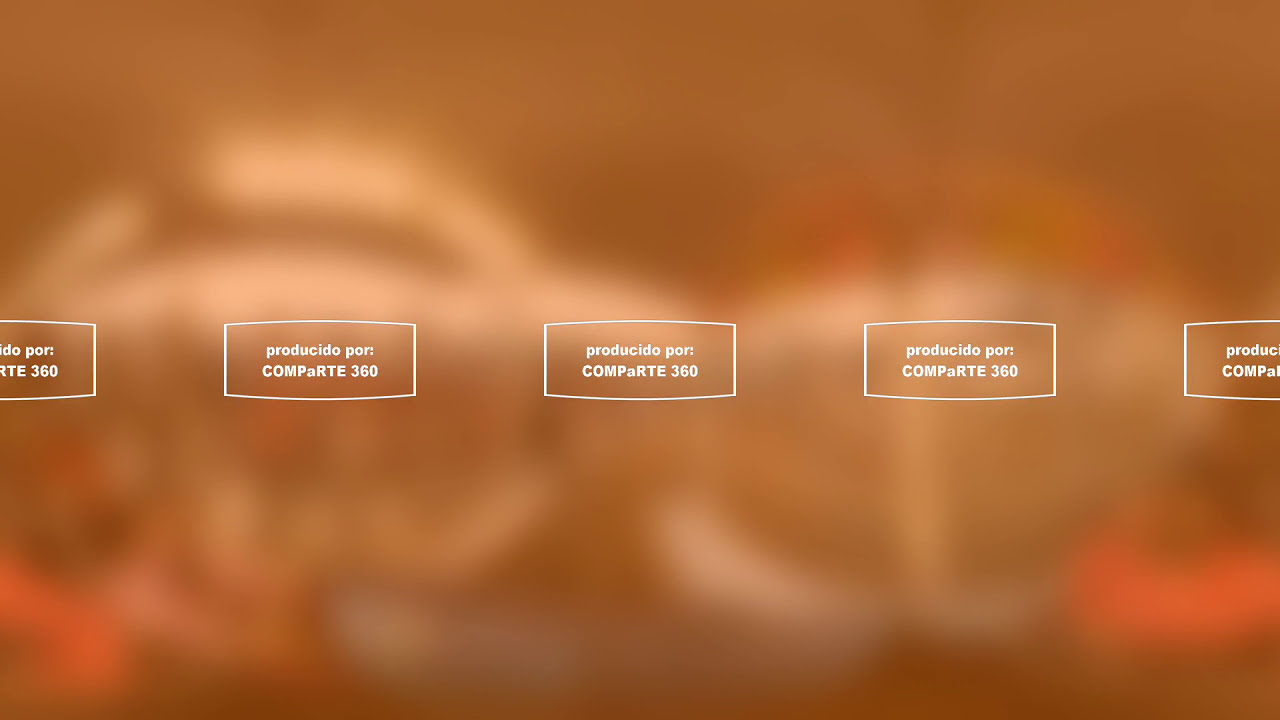The image features a heavily blurred background with a blend of oranges, yellows, whites, and browns, creating a somewhat abstract and indistinct setting. There are five white-bordered rectangular boxes superimposed on this background, each containing text in Spanish. Three central boxes are fully visible and read "Productio Por Comparte 360," while the boxes on the far left and right are partially cropped but appear to display the same text. The text is varied in capitalization, with "ProducioPort" in lowercase and "Comparte360" in a mix of upper and lowercase. The photo's abstract nature—possibly edited with Photoshop—elicits interpretations of it being an animal or something unidentifiable.